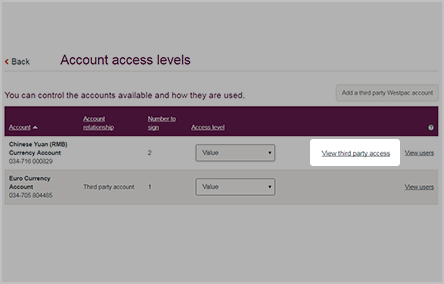This image is a carefully cropped, translucent-overlay screenshot from a web page, specifically focusing on a small but significant section of its content. The visual emphasizes a red back arrow accompanied by the word "Back," suggesting navigational elements. Dominating the scene is a purple-titled header that reads "Account Access Levels."

Beneath this header is a detailed table that outlines various aspects of account management for what appears to be a banking or financial service. The table provides control over account availability and usage, featuring five meticulously labeled columns: "Account," "Account Relationship," "Number to Sign," "Access Levels," and "Option to View Users." Notably, the table includes accounts denominated in Chinese Yuan and Euros, highlighting the platform's international reach.

A distinct feature of the screenshot is a pop-out section detached from the translucent overlay, which is a hyperlink leading to "View Third Party Access."